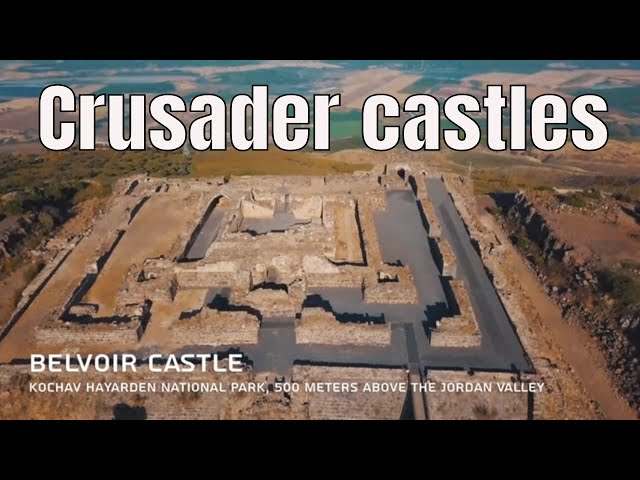The image depicts the remnants of an ancient Crusader castle known as Belvoir Castle, located 500 meters above the Jordan Valley in Kochav Hayarden National Park. The photograph is presented in a widescreen format with black letterbox bars at the top and bottom, giving it a cinematic feel. The castle itself is a large, squared-off structure built with gray stone bricks, now reduced to towering walls and foundational remnants scattered across brown dirt. Surrounding the castle, the landscape features hilly, green rolling areas, with mountains, trees, and valleys descending into what appears to be farmland and sagebrush areas. The bold white text with black borders overlaying the image provides the labels: "Crusader Castles" at the top and "Belvoir Castle, K-O-C-H-A-V-H-A-Y-A-R-D-E-N National Park, 500 meters above the Jordan Valley" at the bottom.